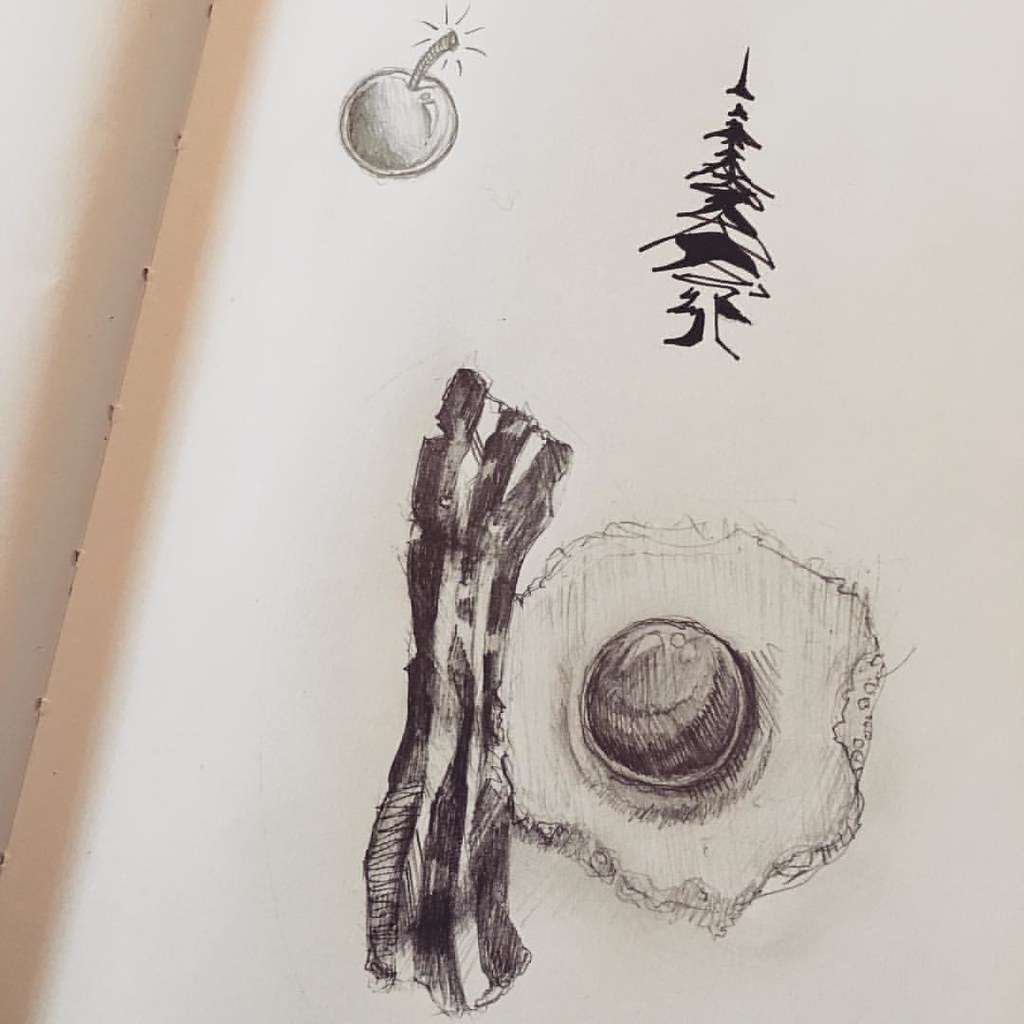This image is a photograph of a pencil and ink drawing on white paper from a sketchbook. The paper shows a slight shadow or discoloration where it was removed from the book, with small holes at the edge where it was held together by string. In the upper left corner, there is a detailed pencil drawing of a cherry with a stem and eight lines radiating from the top, giving it the appearance of a shiny piece of fruit. Some descriptions suggest it might be a more abstract depiction, potentially even resembling a bomb's fuse. To the right of the cherry is a dark, ink-drawn pine tree, resembling a conifer. Below these images, there is a larger pencil sketch of a sunny-side-up egg accompanied by a single strip of bacon, drawn in black and gray tones.